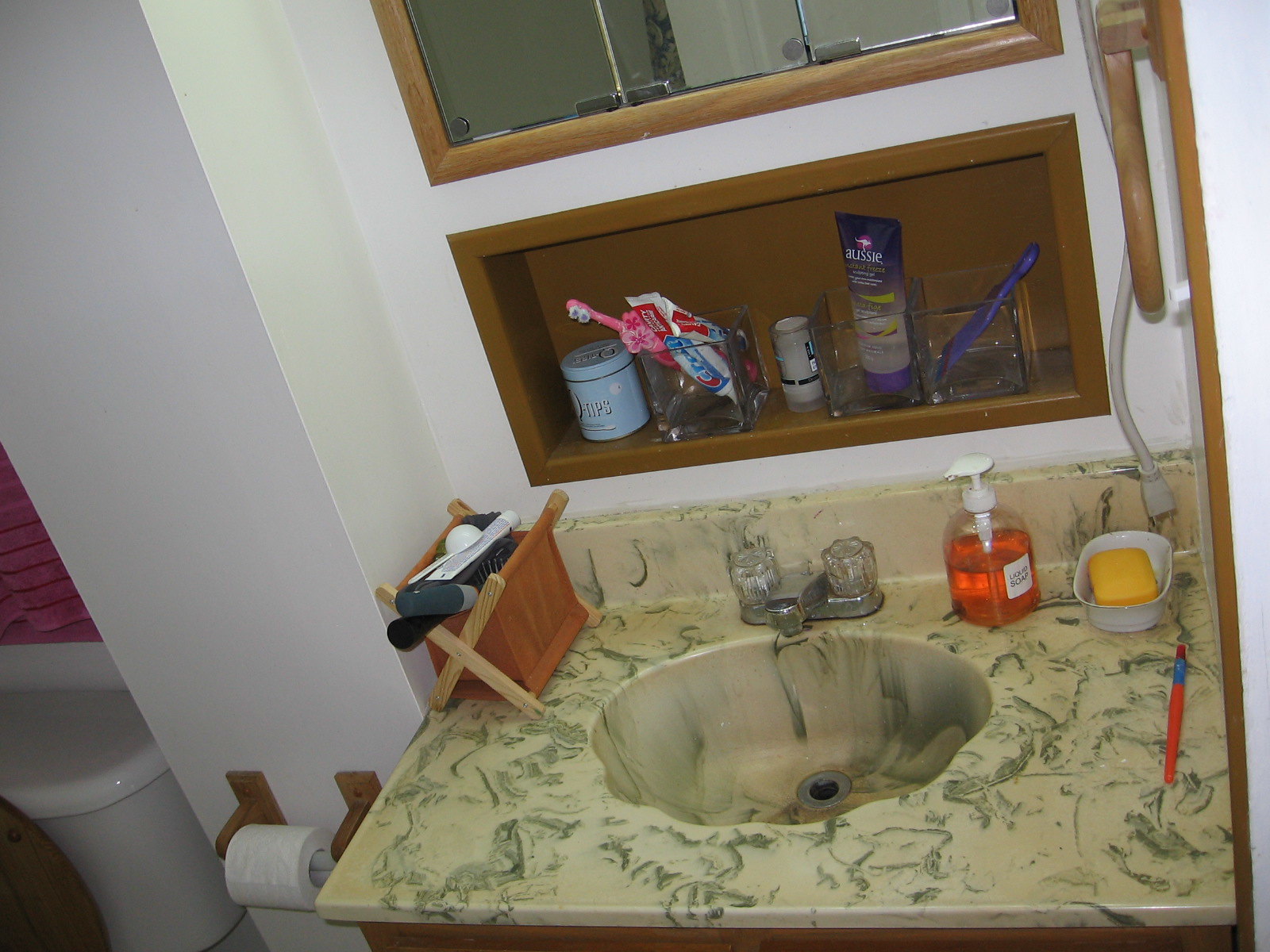This detailed image captures a close-up view of a small bathroom. On the left-hand side of the image, a white wall features a window adorned with pink curtains, patterned with horizontal lines, partially cut out of the frame. Below the window, a white toilet is visible, equipped with a light wooden seat, only the right side of which is visible due to the framing. Adjacent to the toilet, a wooden toilet paper holder is mounted on the wall, holding a roll of white toilet tissue.

Moving further right, we see a bathroom sink with a striking yellow countertop, accented with green, marble-like squiggly lines. Placed on the sink's right side is a red and blue toothbrush, accompanied by an oval-shaped white soap dish containing a yellow bar of soap. Nearby, there is an oval-shaped, clear liquid soap container, labeled "Liquid Soap" in black text on a white square label, with a white nozzle.

Above the sink are the clear, round faucet knobs and a silver water faucet. To the left of the sink, clear, square bins neatly organize various bathroom items. These include a pink toothbrush with floral decorations, two tubes of Crest toothpaste in red, blue, and white packaging, and a purple-tubed hair product. Additionally, a purple hair pick is also visible, rounding out the array of personal care items in this tidy and colorful bathroom scene.